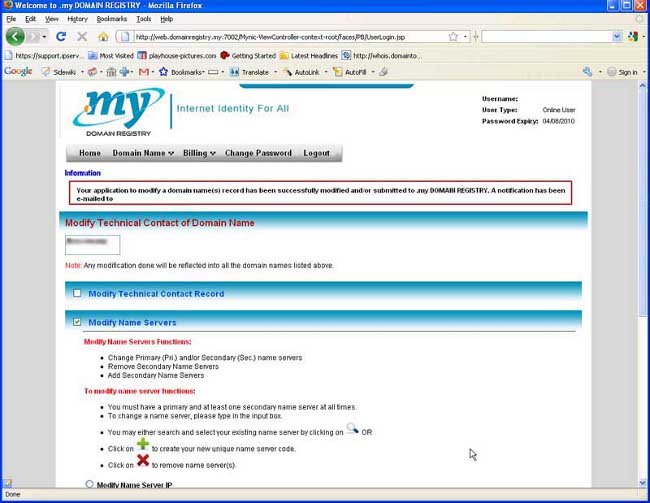In this image, an older version of the Mozilla Firefox browser is displayed. The browser is open to a website titled "My Domain Registry." Prominently displayed in the top left corner of the page is a circular logo featuring the letters “MY,” accompanied by swirling lines. To the right of the logo, the words "domain registry" are written in red, followed by a teal horizontal line that transitions into the phrase "internet identity for all." 

Above the website content, the Firefox browser's interface appears noticeably dated, showcasing elements such as the favorites bar, search bar, and standard navigation buttons like refresh, close, back, and home. Traditional menu options like file, edit, and view are also visible, evoking a sense of nostalgia for previous browser designs.

Directly below the MY symbol are navigational links for different sections of the website, including home, domain name, billing, change passwords, and logout. The main body of the page displays a notification stating, “Your application to modify a domain name record has been successfully modified and/or submitted in My Domain Registry and a notification has been sent.” This message indicates that the user recently submitted a request related to domain name management. Further options for modifying the server are listed below the notification, though they are not detailed in the description.